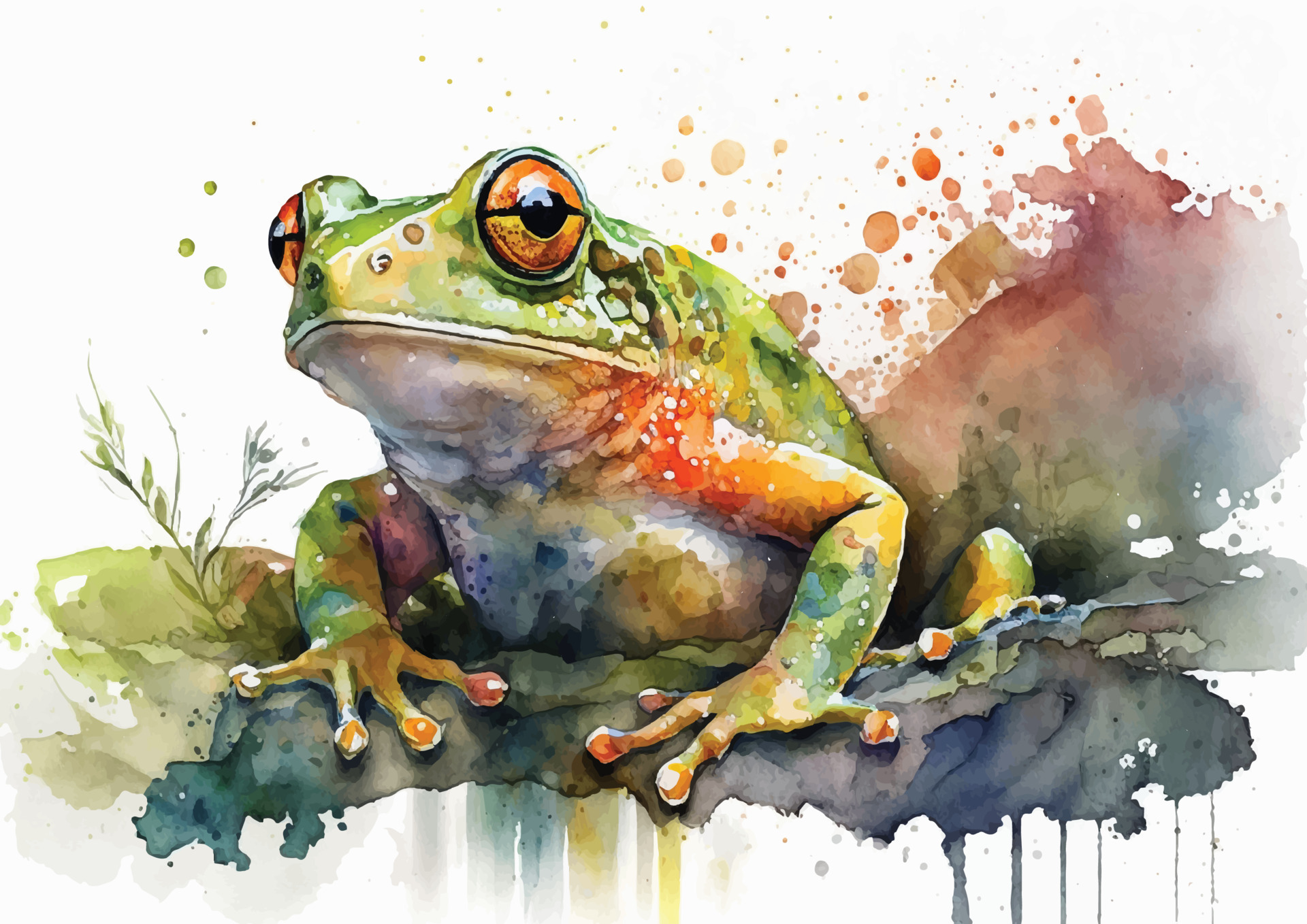The detailed watercolor painting features a predominantly green frog perched atop a colorful, abstract palette of paint blotches. The palette transitions from lime green and deep green to blues and vibrant yellows at the center, with the colors dripping downwards and blending into reds and oranges on the right side near the top. The frog itself, primarily green, exhibits a mix of other vivid hues including orange, red, and yellow, particularly noticeable around its arms and the four-fingered extremities. The frog's eyes are distinct with a striking orange color bisected by black horizontal pupils, and it displays a plain, contemplative expression as it gazes off to the side. The white underbelly of the frog is accented with patches of blue and yellow, adding to its detailed texture. Surrounding the frog, the background is filled with various paint splatters and drips, with significant black and red splotches to the right. Additionally, there is a single tall blade of grass situated under its left arm, enhancing the overall naturalistic yet abstract composition of the painting.